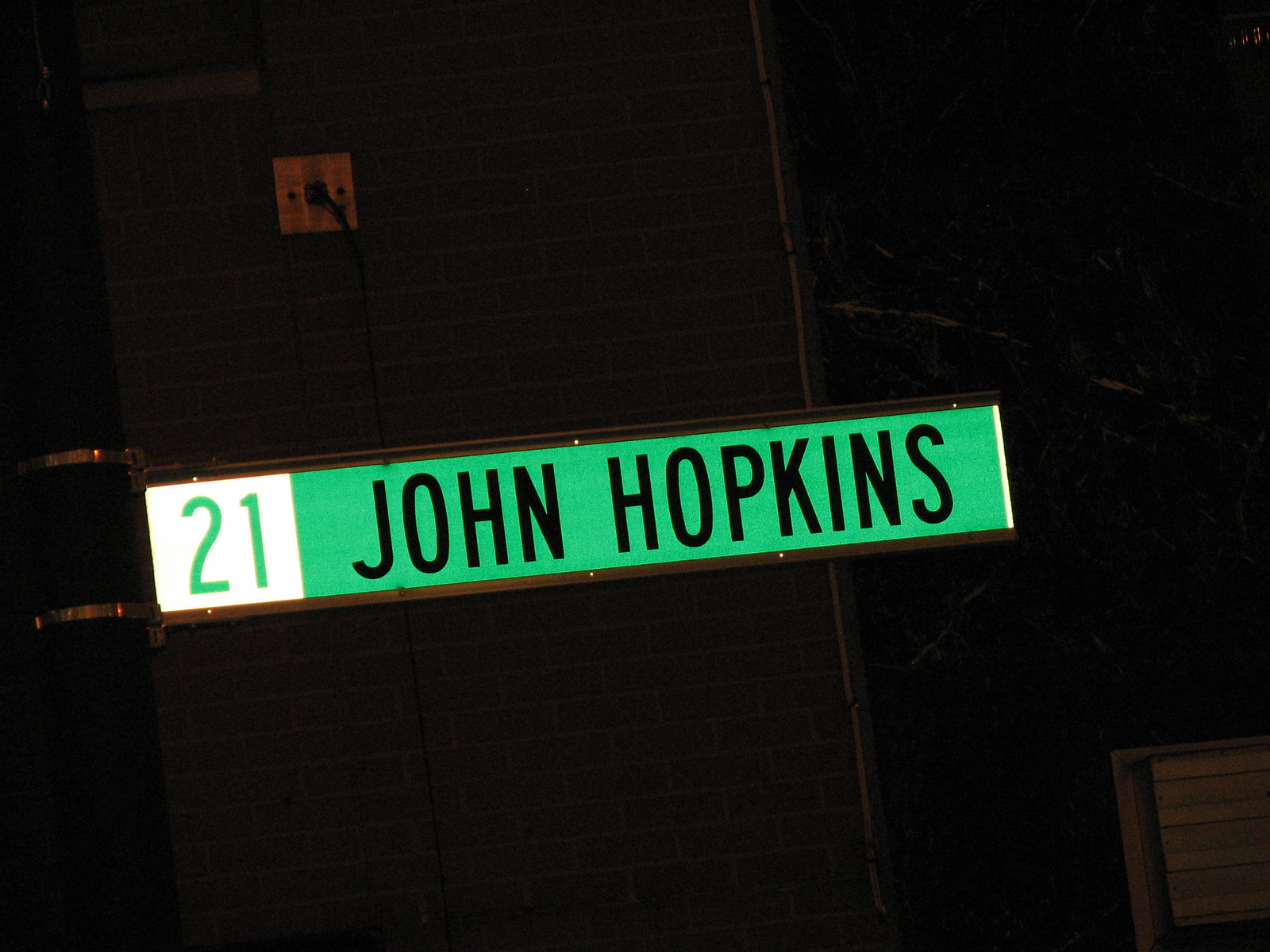The photograph, taken at night, captures the facade of a stone building accentuated by white grout lines. In front of the building stands a prominent black pole adorned with a silver metal band. Attached to this pole is a tricolor sign in black, white, and green, displaying "John Hopkins" in black font over a green background and the number "21" in green off to the side. Behind the sign, a black cord-like structure can be seen running down the front of the building. In one corner of the image, a white, square object with gray shadowing is partially visible. The majority of the image is enveloped in darkness, rendering additional details difficult to discern. Despite the low light, the photograph maintains a decent quality.